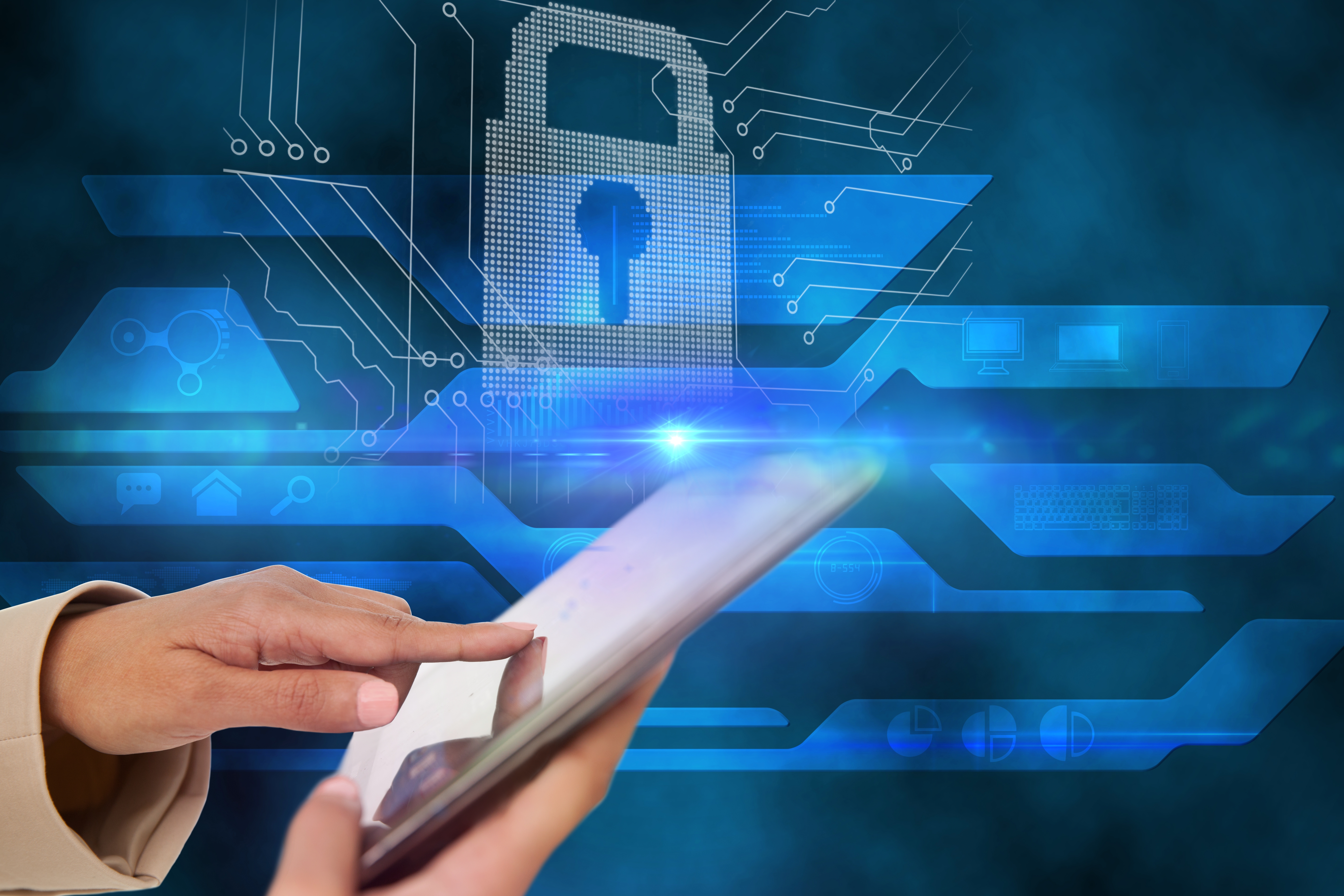This digital poster prominently features the hands of a person engaging with a touch screen tablet, viewed from the side. The left hand, which has light-colored skin and pink nail polish, suggests it might be a female, and it is delicately using its pointer finger to interact with the tablet. The right hand firmly holds the device, which is potentially a larger version of a smartphone or tablet. The person's wrists are adorned with the sleeves of a cream-colored or beige coat, indicating a sense of elegance.

The background exudes a high-tech, cyber security theme, primarily in shades of blue, ranging from dark to light hues. The backdrop showcases intricate digital lines and geometric shapes that create an engaging, futuristic aesthetic. A prominently featured digital lock, complete with a keyhole, underscores the theme of security. This lock is surrounded by bright lines and schematics reminiscent of a circuit board, reinforcing the cyber security motif of the poster.